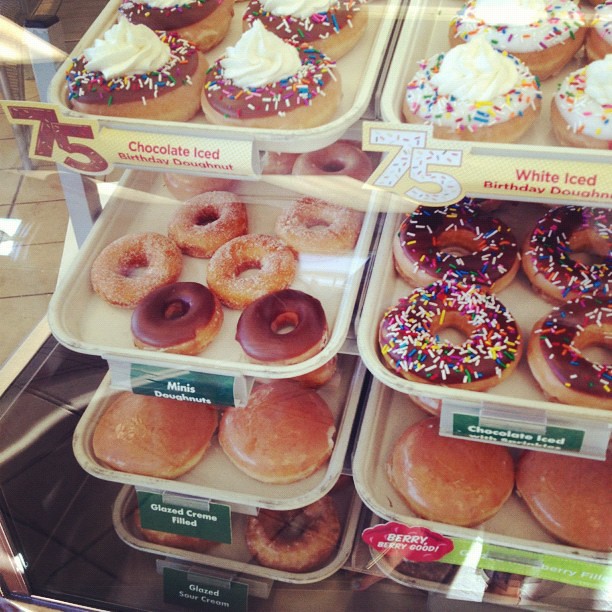This is a color photograph capturing a bakery display case filled with a variety of doughnuts arranged on four shelves. The top row features chocolate-iced birthday doughnuts on the left and white-iced birthday doughnuts on the right, all adorned with festive sprinkles and a large mound of icing in the center. Moving to the second row, there are mini doughnuts on the left side, followed by chocolate-iced doughnuts with sprinkles. The third row down showcases glazed cream-filled doughnuts. At the bottom layer, additional cake doughnuts and yeast doughnuts with a sugar glaze can be seen, adding to the delectable assortment within the transparent, glass-fronted display case.